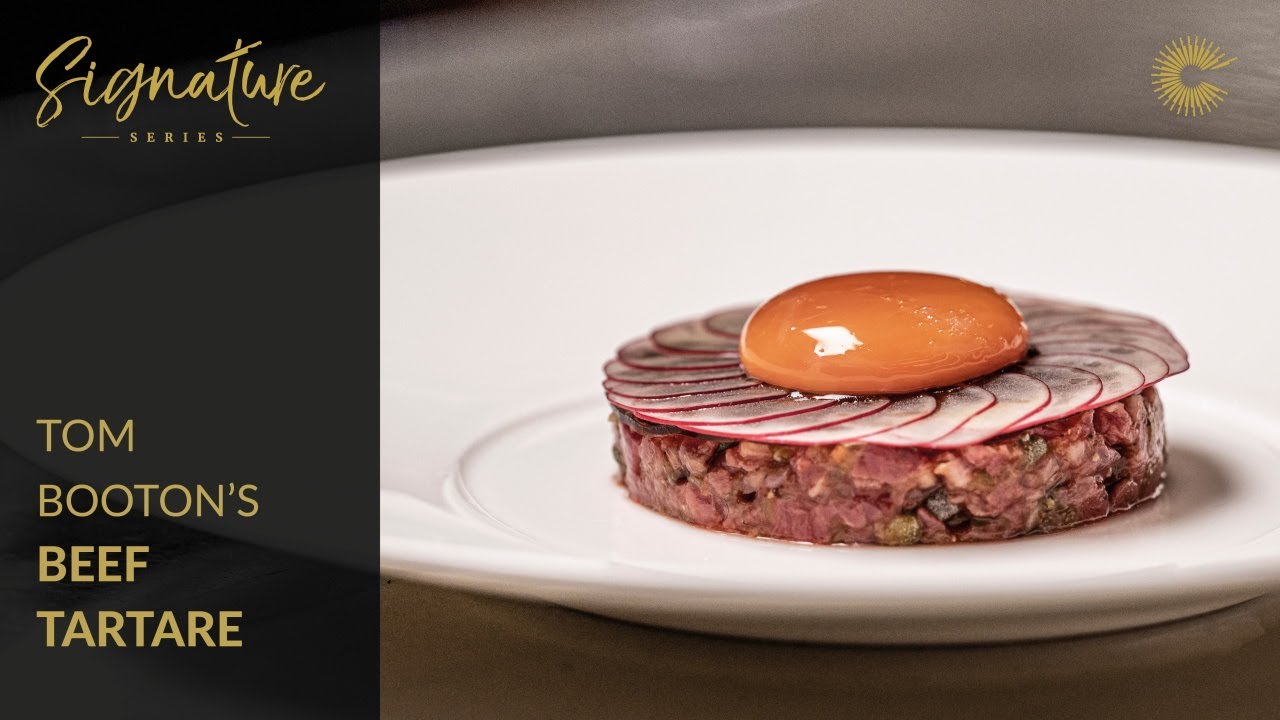This indoor photograph captures a close-up of a white plate showcasing Tom Booten's signature dish: Beef Tartare. The dish features a raw beef patty, intricately mixed with vegetables including green peppers and possibly chopped black olives. Atop the beef, very thinly sliced radishes are arranged in a fan shape, radiating elegantly. Crowned in the center of the radishes is a dark tan, shiny egg yolk. On the left side of the image, the black vertical rectangle prominently displays gold text reading "Signature Series" in cursive, with "Tom Booten's Beef Tartare" beneath it in bold. In the top right corner, a gold logo shaped like a 'C' crafted from butcher knives adds a final touch of sophistication. The white plate rests on a reflective brown table, enhancing the dish’s presentation.